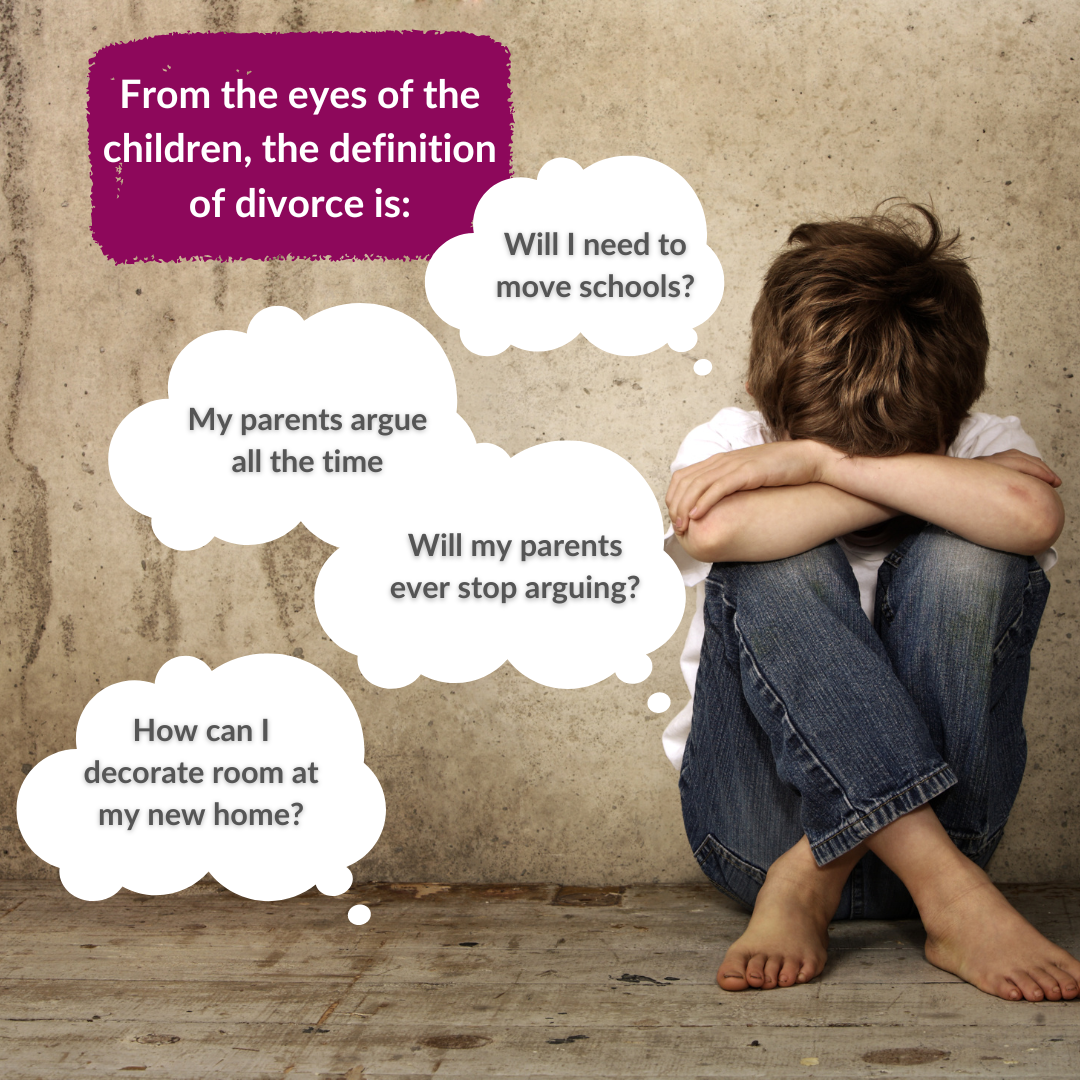The image depicts a young boy with blondish-brown messy hair, sitting on a dirty concrete floor with a similarly grimy wall behind him. He is dressed in blue jeans, a white t-shirt, and is barefoot, his feet showing signs of dirt. The boy is hunched over in a fetal-like position, with his knees drawn up to his chest and his head resting on his forearms, which are braced on his knees. He has a small bruise on his elbow. The mood of the image is somber, highlighting the emotional turmoil children face during divorce.

In the upper left-hand corner, a purple rectangular box contains white text that reads, "From the eyes of children, the definition of divorce is." To the right of this text, several white cloud-shaped thought bubbles with black writing emanate from around the boy's head, expressing his distressing thoughts: "Will I need to move schools?", "My parents argue all the time.", "Will my parents ever stop arguing?", and "How can I decorate my room at my new home?" The combination of the boy's posture and the text effectively communicates the anxiety and uncertainty children often experience during their parents' divorce.